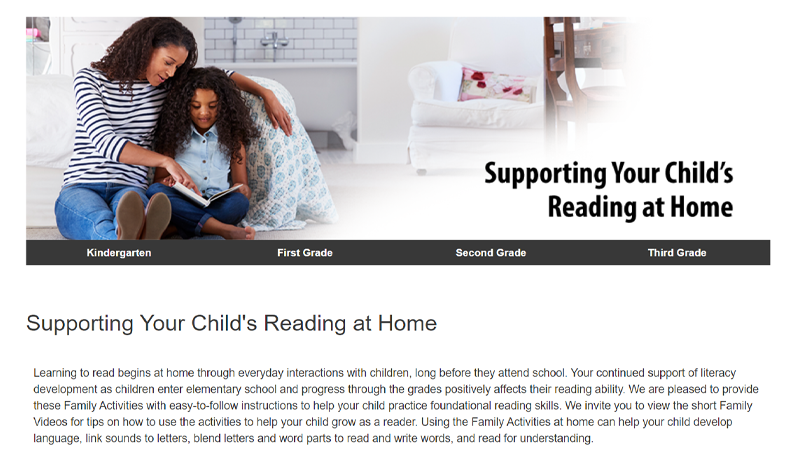This is a screenshot of a website dedicated to supporting children's reading at home. The top section of the webpage features a heartwarming photograph of a woman and her child seated in a cozy room, engaged in reading a book together. The woman is actively assisting her child in the reading process. Stretching across the middle portion of the page is a distinctive black banner with white text showcasing navigational links labeled "Kindergarten," "First Grade," "Second Grade," and "Third Grade" to guide users to specific sections catered to different educational levels. Directly below the banner, there is a prominent white area containing black text. This text emphasizes the foundational role of early reading experiences at home, stating, "Learning to read begins at home through everyday interactions with children long before they attend school. Your continued support of literacy development as children enter elementary school and progress through grades positively affects their reading ability."